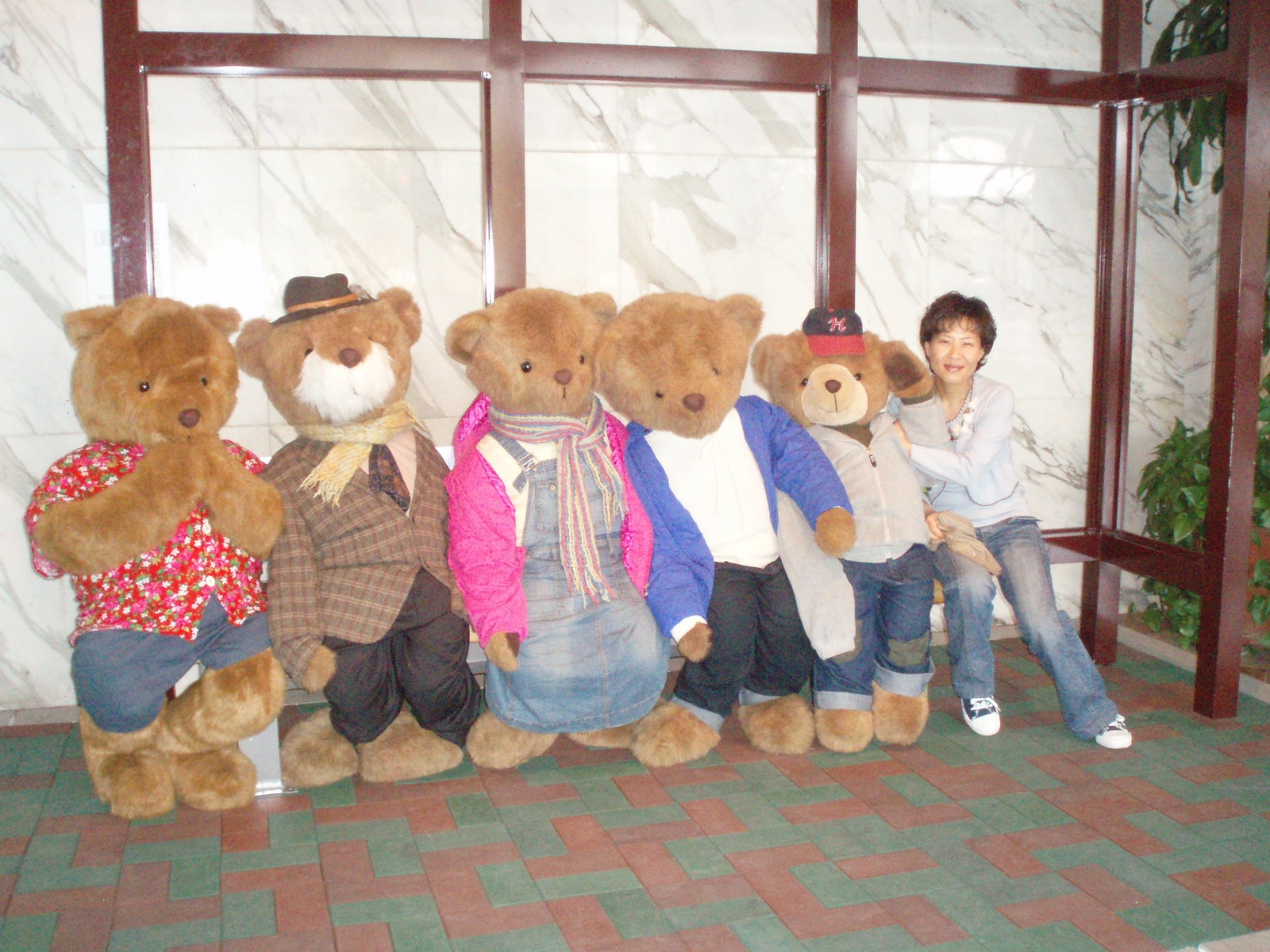This detailed color photograph captures an Asian woman with short, dark hair, seated on a wooden bench. She's wearing blue jeans, white and black sneakers, and a light-colored, long-sleeve gray sweater. The bench is placed against a wall that looks like it is made from marble. Seated next to the woman are five gigantic teddy bears, each donned in unique outfits and as tall as the seated woman. The first bear is dressed in a baseball cap, a cardigan, and jeans. The second bear sports a blue sport coat. The third bear is outfitted in a dress made from overalls and a pink parka. The fourth bear wears a plaid suit coat and a brown fedora. The fifth and final bear is clad in a short-sleeve camp shirt, with its hands posed as if in prayer. All the bears have light brown, golden fur. The floor beneath them features a green hue with brown L-shaped patterns. The backdrop combines the wooden frame of the bench and a distinct marble-like wall, adding a unique juxtaposition to the scene.